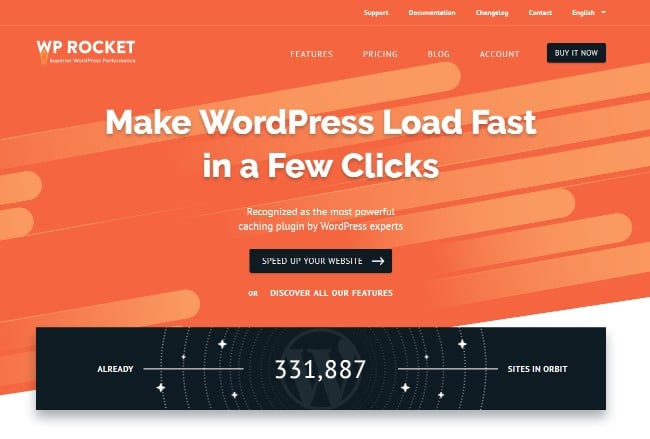The image is a screenshot of a website page for WP Rocket, a caching plugin for WordPress. At the top of the page, there is a navigation bar that includes the links: "Support," "Documentation," "Change Log," "Contact," and a language option labeled "English." Below this, another row features links to different sections of the site: "Features," "Pricing," "Blog," and "Account," followed by a prominent black button with white text that reads "Buy It Now."

The background of the website has a vibrant orange hue, with a pattern of slightly lighter, thick, two-dimensional lines running through it. This creates a visually appealing design that is both modern and dynamic. Across this orange background, in large, white text, the headline announces, "Make WordPress Load Fast in a Few Clicks." Beneath this, smaller white text proclaims, "Recognized as the Most Powerful Caching Plugin by WordPress Experts." Further down, another black button with white text urges visitors to "Speed Up Your Website." Overall, the design is clean, colorful, and centered around conveying the efficiency and power of the WP Rocket plugin.